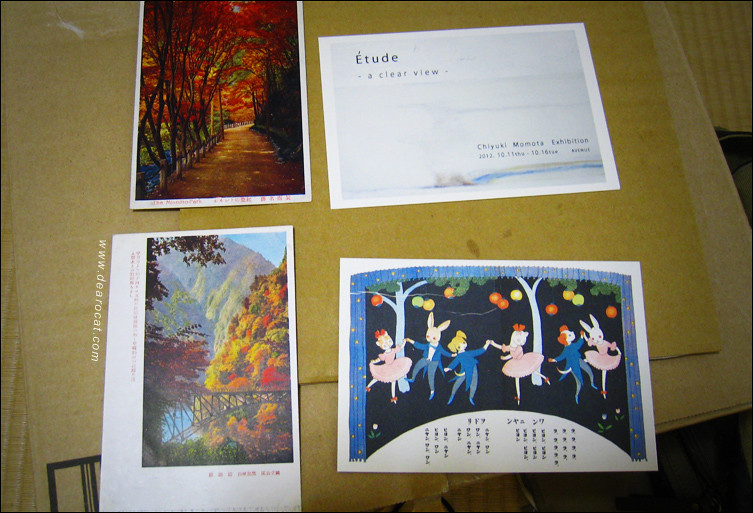This overhead color photograph captures a top-down view of a light tan to grayish-colored table surface, arranged with four distinct postcards. The upper left postcard is a partial image showing a road winding into a vibrant fall scene framed by trees in autumnal hues. Beside it, oriented landscape, is a predominantly white postcard that reads "Etude: A Clear View, Chiyuki Momota Exhibition" in black lettering. The lower left postcard features a serene nature scene of a railroad bridge arching over a deep ravine with surrounding mountains blanketed in fall foliage. Adjacent to this, in landscape orientation on the lower right, is a whimsical sketch of animals dressed in formal attire—rabbits, dogs, and cats—dancing under trees against a black backdrop. Japanese text on the bottom right postcard and a web address, www.dearocat.com, provide further intrigue to the collection.